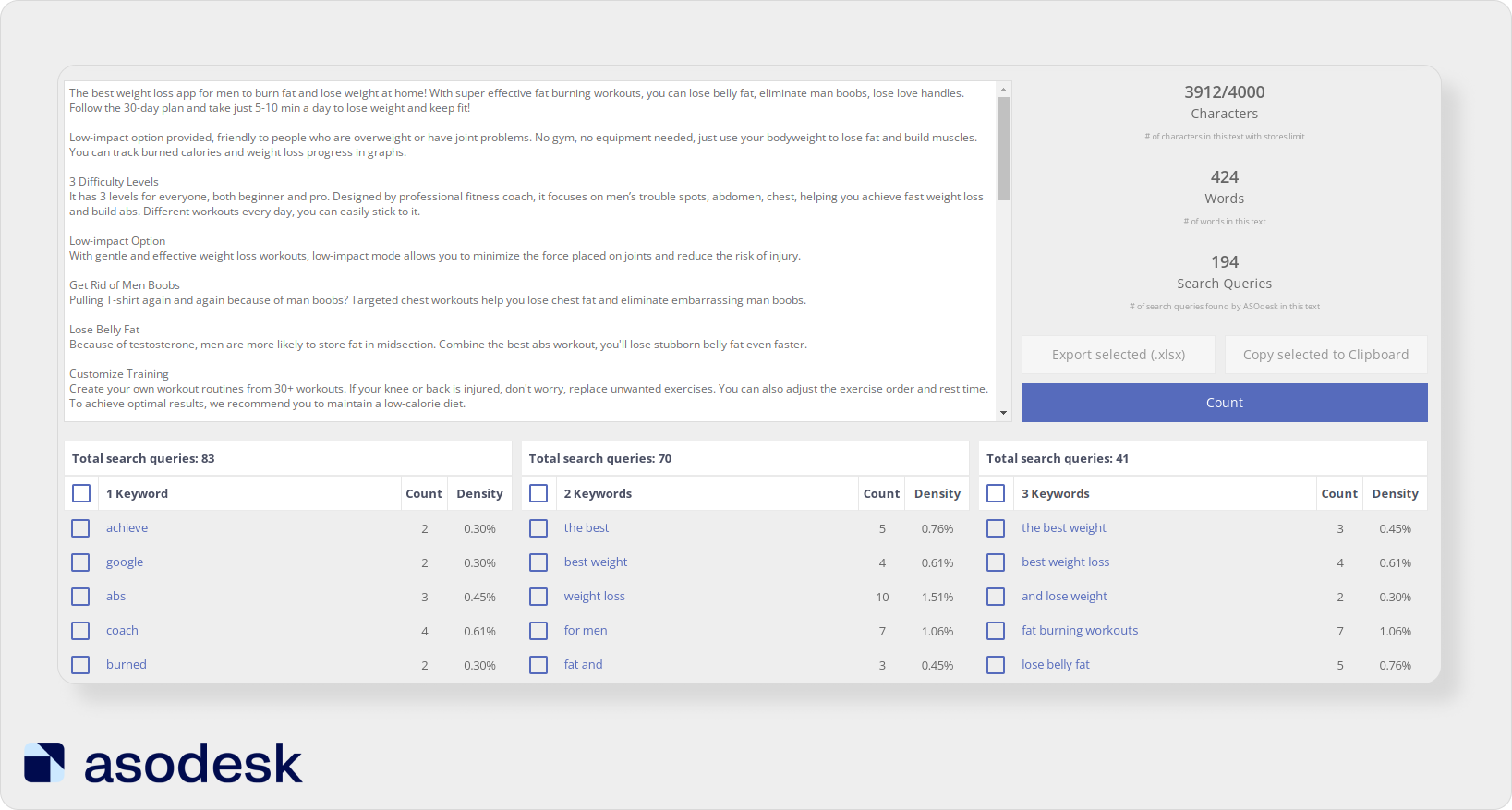This screenshot displays the interface of the ASO Desk platform, characterized by a light gray background. Situated in the bottom-left corner is a distinctive logo: a dark blue square within a light blue square, accompanied by the text "ASO desk" rendered in dark gray lowercase letters.

Prominently featured in the top-left segment is a large text box containing several lines of black text on a white background, although the text is not legible. Adjacent to this, on the right, various metrics and data points are displayed. Specifically, it notes "3,912 out of 4,000 characters," followed by "424 words," and "194 search queries," with additional small, unreadable lines of text appearing beneath each metric.

Below these metrics are three action buttons: the top two being white and positioned side-by-side, labeled "Export selected .xlsx" and "Copy selected to clipboard," respectively. Beneath these is a larger blue button labeled "Count."

Further down the interface, a section with three columns is visible. While the contents of these columns are not legible, they likely display different metrics or data sets. Each column appears to have a top line marked "Total search queries," followed by different numerical values. The detailed content of these sections remains unclear.